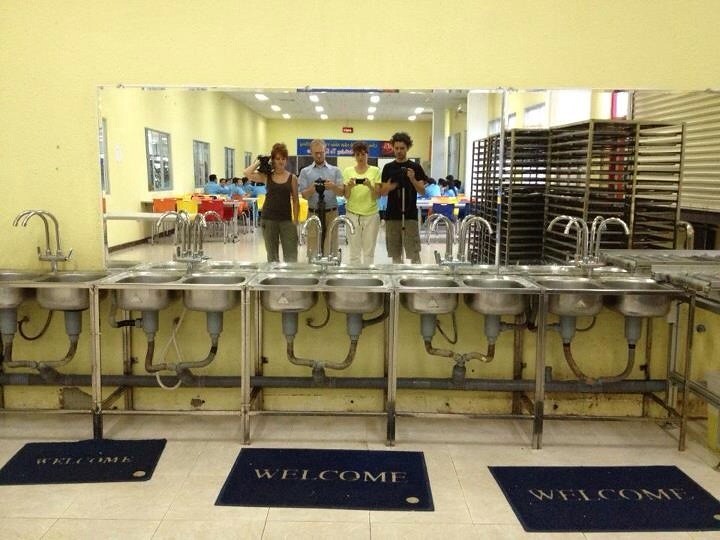The photograph depicts an industrial-like setting, possibly a cafeteria or food prep area, characterized by a long rectangular mirror spanning almost the entire yellow back wall, with the exception of a small metal square on the left. In front of the mirror, five double-sided sinks with exposed piping underneath are visible, creating an industrial ambiance. Four people—two women and two men—stand aligned in front of the mirror, each taking photos or videos with their phones. The individuals are dressed distinctively: the woman on the left wears a black tank top, followed by a man in a blue office shirt and khakis, then another woman in a bright yellow shirt with white pants, and finally, a man in a black shirt and cargo shorts. The floor beneath their feet features three black welcome mats with cream-colored text, set against a light gray marbled tile. In the reflection, there are various colored chairs—red, yellow, orange, and blue—alongside people in blue shirts who appear to be engaged in an activity, potentially a class. Additionally, commercial racks for cooling baked goods are visible to the right, adding to the industrial kitchen aesthetic.